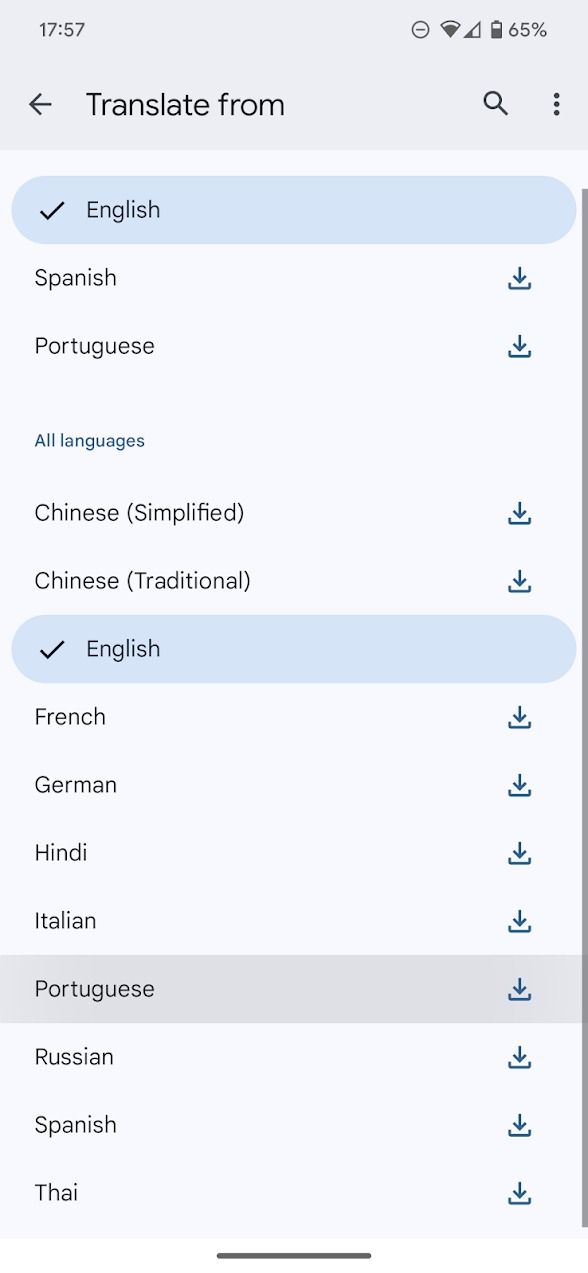This screenshot captures the translation configuration settings on a smartphone application. At the top of the screen, the status bar displays essential information including the current time, battery level, and signal strength. Below this, the interface highlights the translation menu where users can select languages for translation.

The title "Translate From" indicates the feature's function, prompting users to choose a source language from a comprehensive list. The listed languages include English, Spanish, Portuguese, Chinese Simplified, Chinese Traditional, French, German, Hindi, Italian, Portuguese, Russian, Spanish, and Thai. Currently, English is selected, as indicated by a checkmark beside it.

Each language entry features a download icon on the right, which allows users to download the language for offline use. Notably, the languages that have already been downloaded (such as English, in this instance) do not display the download icon, signifying their availability for immediate use without requiring an additional download.